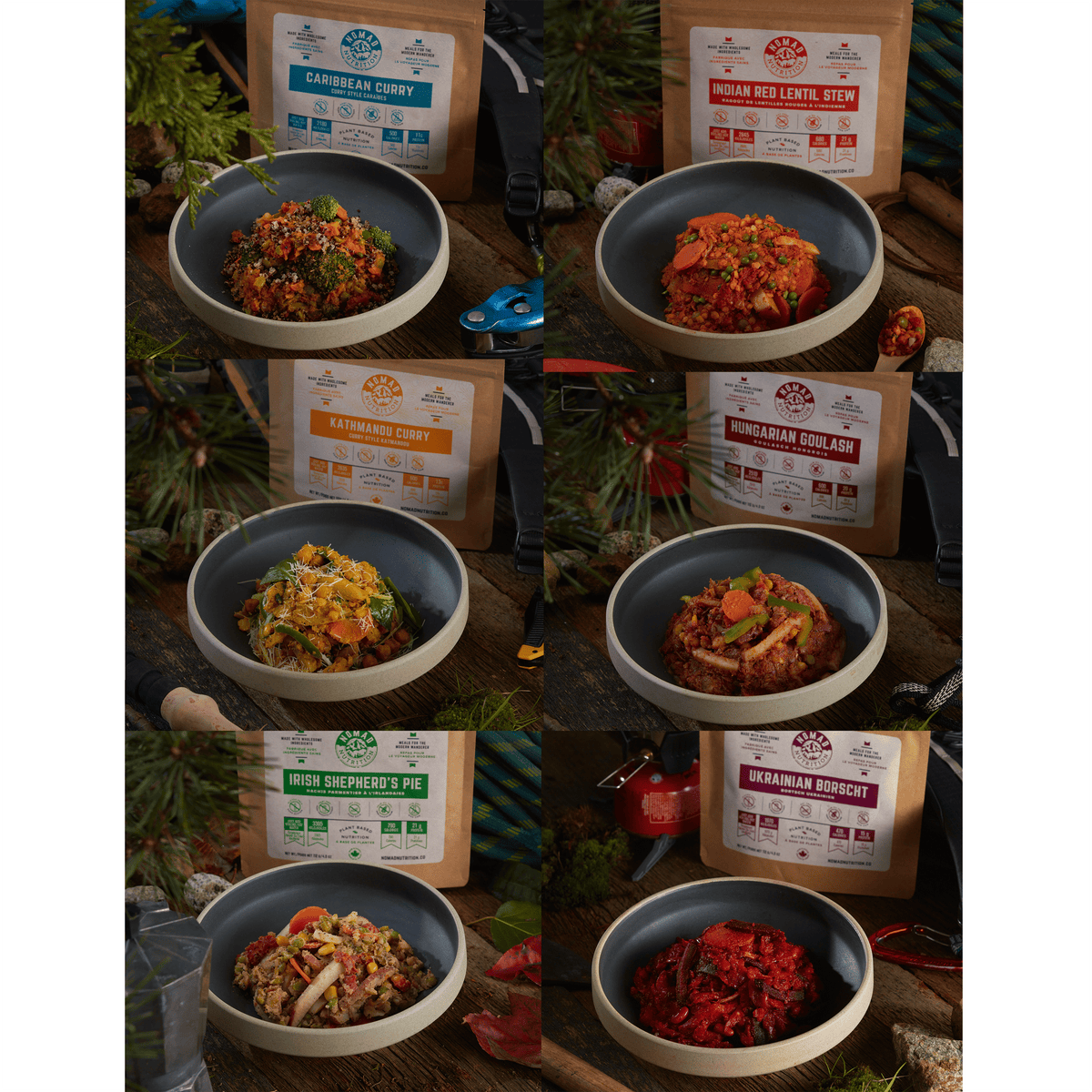The image shows six distinct bowls of prepared food, each representing different prepackaged meals. These bowls are displayed in a vertical rectangle layout, arranged in two columns of three photographs each. Each bowl is positioned on a dark wooden surface, likely a deck or bench, with greenery and sprigs from trees and plants in the background. 

Behind each bowl, there is a light brown rectangular baggie with a rustic, white label containing colored text that names the dish inside. The bowls themselves have a white exterior and a black interior, creating a visually appealing contrast. 

The dishes showcased are:
1. Caribbean Curry – Featuring rice, broccoli, and possibly meat, the dish looks spicy with a mix of vibrant colors.
2. Indian Red Lentil Stew – Characterized by a reddish color with slices of red, green capers, or peas mixed in.
3. Katmandu Curry – A yellowish-hued dish.
4. Hungarian Goulash – Though not detailed in the voice captions, it is among the displayed foods.
5. Irish Shepherd's Pie – Also not elaborately described but is present in the spread.
6. Ukrainian Borscht – Noted for its dark red color.

Each bowl and its corresponding baggie are designed to visually communicate what the prepared food will look like, emphasizing the variety and appeal of these prepackaged meals.